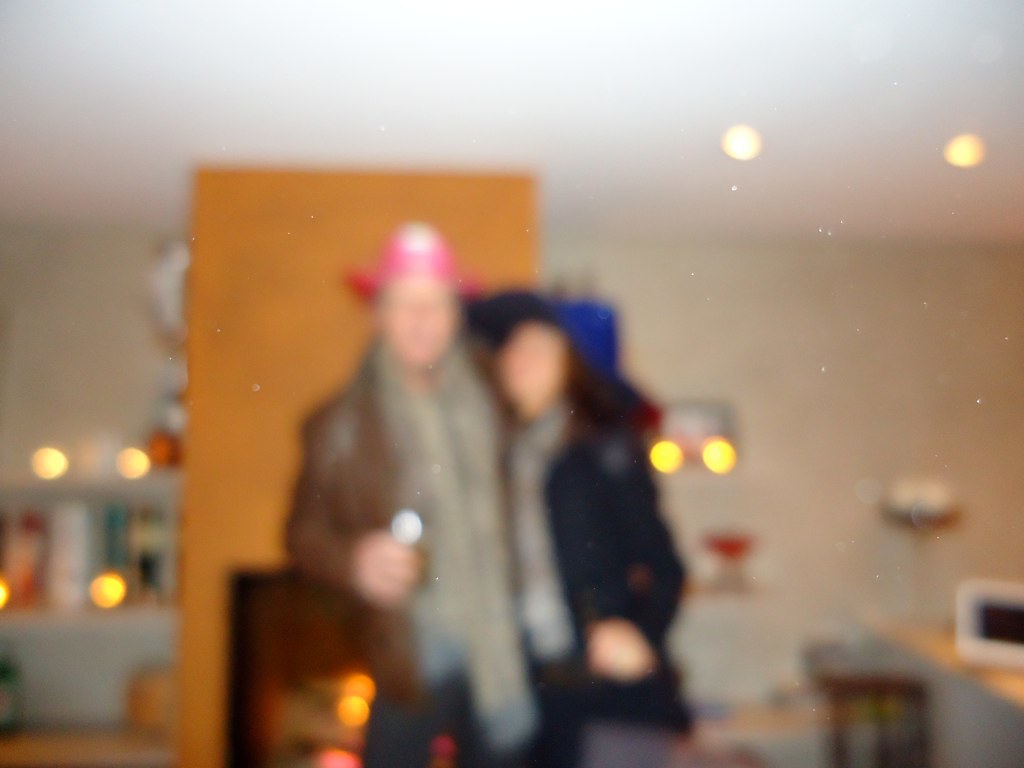A slightly blurred photograph captures a cozy indoor moment featuring a man and a woman standing together in a living room. Positioned in front of a fireplace adorned with yellow trim that extends up to the ceiling, the couple appears ready for a casual occasion. The man stands confidently, wearing a whimsical plastic fireman’s cap and draped in a scarf over his brown leather jacket. His attire is completed with blue jeans, and he holds an indistinct object in his hand. Beside him, the woman sports a gray shirt beneath an open black jacket, paired with gray pants. A blue hat adds a playful touch to her ensemble. The white back wall behind them glows warmly with the reflection of little yellow lights, adding to the room's inviting ambiance.